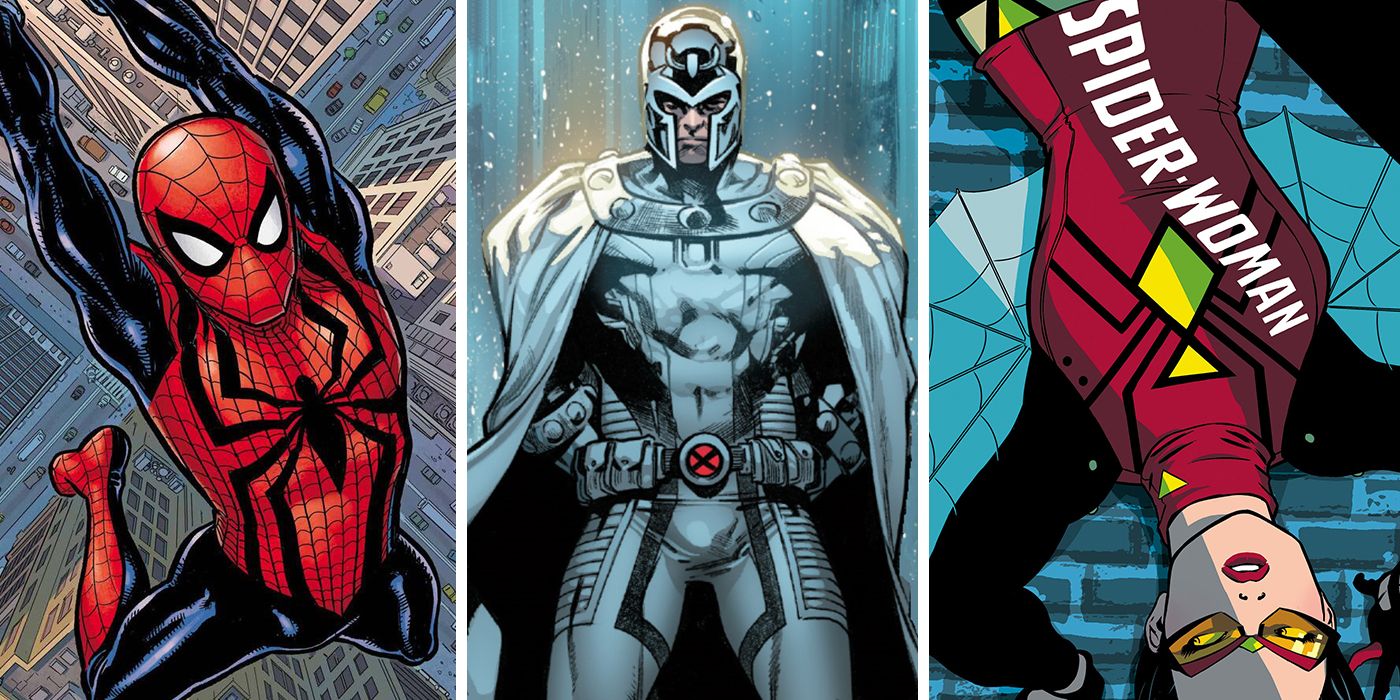The comic book image is divided into three equal panels, each showcasing a distinct superhero. On the far left, Spider-Man is the central focus, depicted mid-swing high above the cityscape. His black and red suit prominently features a black spider emblem on his chest, with matching red mask. The background reveals a dizzying view of buildings and a street far below, dotted with tiny cars, emphasizing his altitude and dynamic motion as he propels himself through the air.

The central panel features a formidable-looking superhero clad in a sleek, metallic silver uniform complete with a knight-like helmet that leaves his face partially visible. He sports a distinctive belt with a red, X-shaped buckle, and a matching silver cape billows behind him. The background is shaded in greenish-silver hues, reflecting the overall futuristic theme of his armor and intense demeanor.

On the right, Spider-Woman is depicted upside-down, with the word "Spider-Woman" prominently displayed on her suit. She wears yellow sunglasses and her suit combines red, yellow, and black colors. Her arms and chest are connected by web-like wings, suggesting mobility through web spinning. The backdrop is a bluish brick wall, further highlighting her unique pose and costume details. The three panels together create a vivid tableau of superhero action and character design.